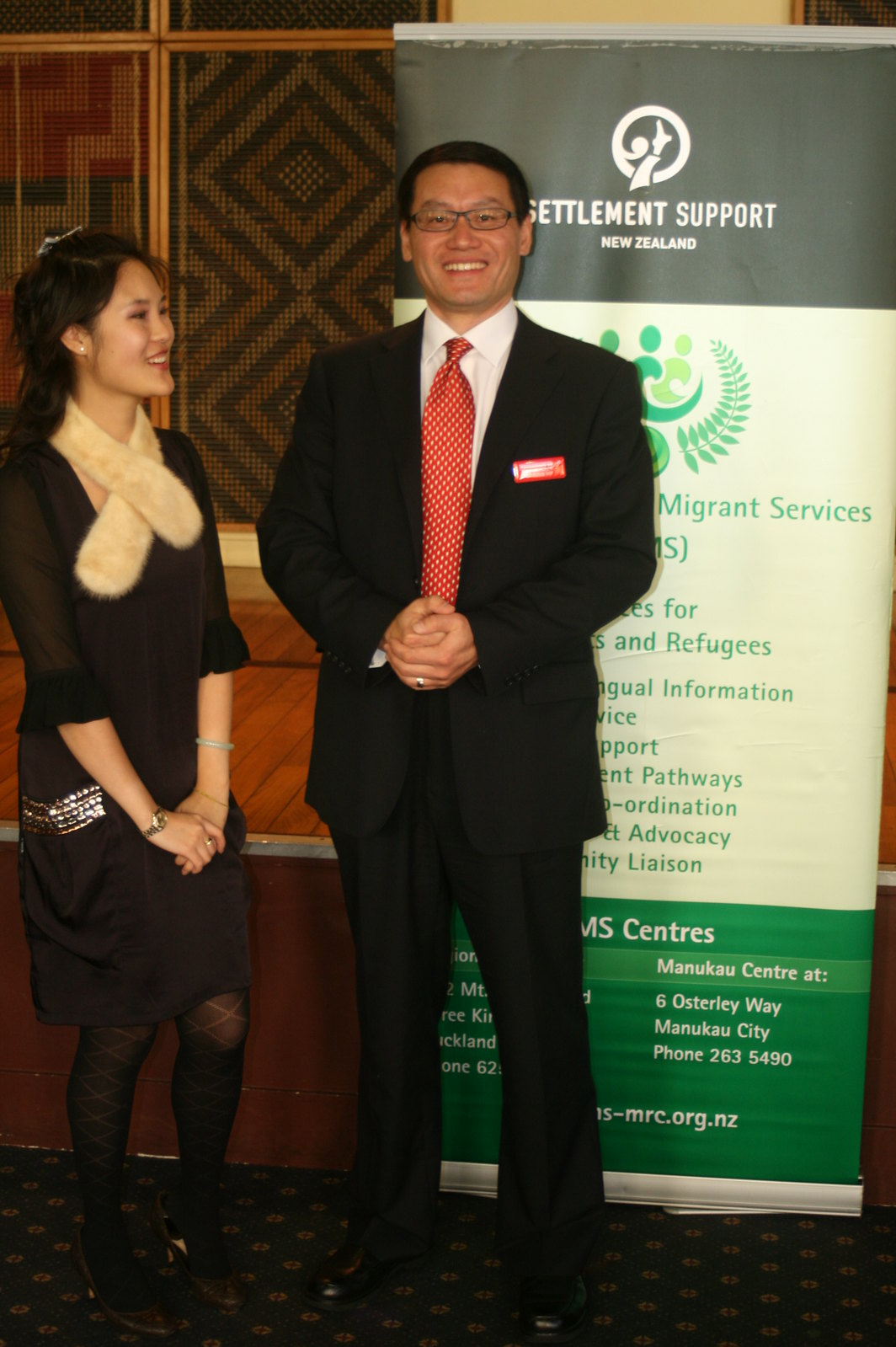The photograph captures a well-dressed young man and woman, seemingly at a conference focusing on settlement support and migrant services, possibly in New Zealand. The woman stands on the left side of the image, her body slightly turned to the right, gazing in that direction. She has shoulder-length dark hair and wears a dark dress, with her hands clasped at her waist. Draped around her neck is what appears to be a fluffy yellow scarf that crosses in front of her chest.

Beside her, the young man faces forward. He has short black hair, glasses, and is dressed in a dark business suit with a white shirt and a red tie adorned with small white dots. His hands are also clasped in front of his waist. Behind them is a large poster or banner that reads "Settlement Support New Zealand" across the top in white letters on a gray background. The poster displays an emblem and various text sections in white and green, along with a website at the bottom.

To the left in the photo is a wall adorned with tapestry-like fabric designs separated by wooden panels. Below this decorative section is a two-toned wooden panel, possibly with the bottom section painted darker. The floor they're standing on is carpeted in a dark color with a gold pattern running through it, completing the formal and professional atmosphere of the scene.